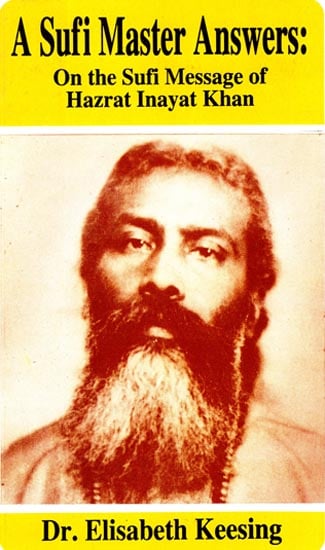This is a color image that appears to be a book cover or a flyer for a program, possibly a lecture. The central feature of the design is a black-and-white photograph of a man with Middle Eastern or Indian descent. The man has short, dark, curly hair, a thick mustache, and a long beard that is graying at the chin. His image, tinted in a sepia-like or reddish tone, is set against a light background, giving the photo a distinct, textured feel. Above the photograph is a yellow band with black text that reads, "A Sufi Master Answers: On the Sufi Message of Hazrat Inayat Khan." At the bottom is another yellow band with black text that says, "Dr. Elizabeth Keesing." The entire layout is framed by a white background, emphasizing the classic and scholarly aesthetic of the design.